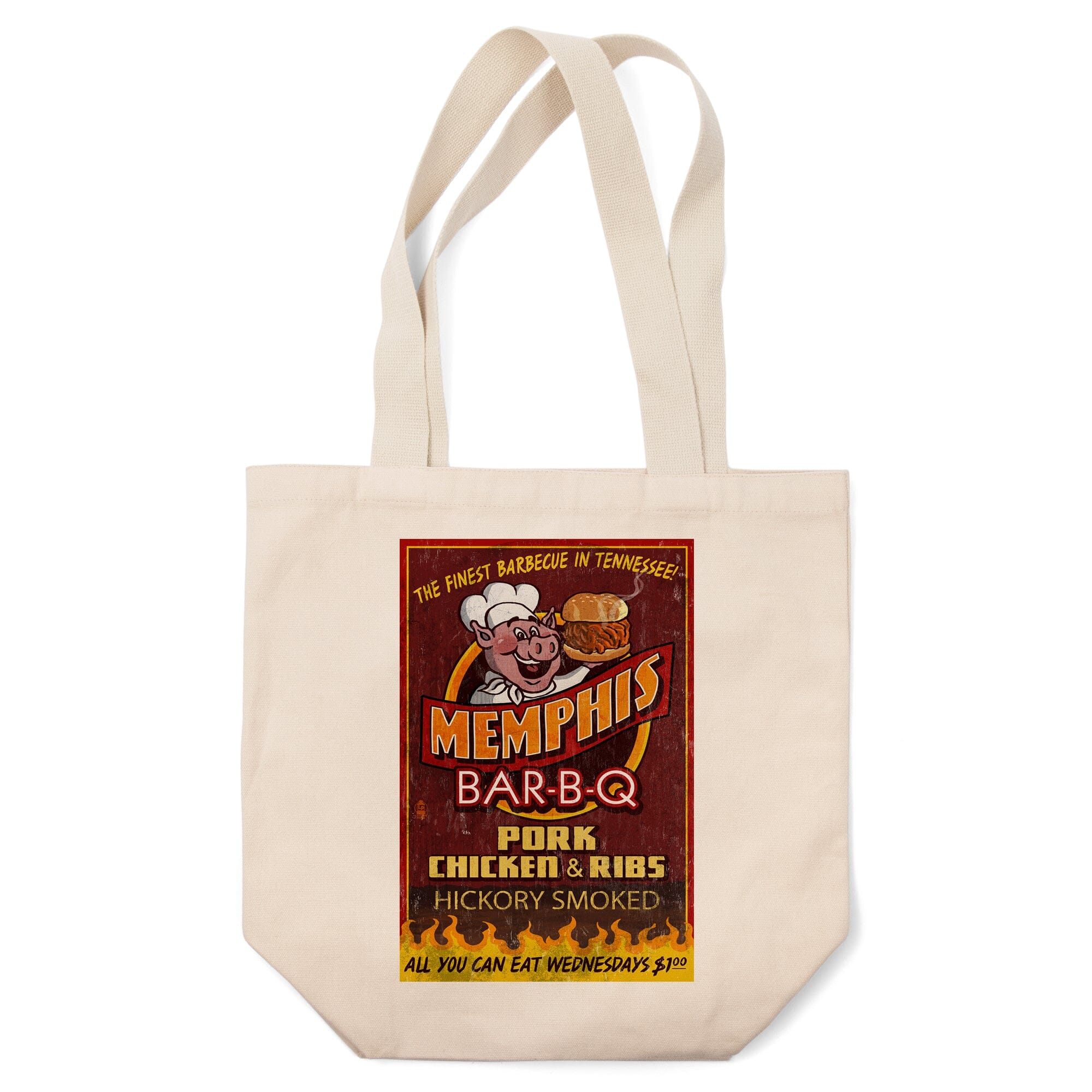This image depicts a cream-colored canvas tote bag lying flat against a white background, presenting a distinct advertisement for a Memphis barbecue restaurant. The tote bag has two slightly curved straps extending from the top corners, and its lower corners are artistically angled. Dominating the center of the tote bag is a rectangular graphic panel with a dark red background and a vibrant circular orange design featuring a cartoon pig dressed in a white chef's outfit, triumphantly holding a barbecue brisket sandwich.

Above the pig, in an arched yellow text, is the phrase "THE FINEST BAR-B-Q IN TENNESSEE!" Below the illustration, the word "MEMPHIS" is prominently displayed in orange, followed by "BAR-B-Q" in a neon effect pink text. Continuing downward, the menu items "pork, chicken, and ribs" are listed in yellow, accompanied by the descriptor "hickory smoked" in smaller white text. The bottom of the graphic showcases yellow flames with black text, advertising "ALL YOU CAN EAT WEDNESDAYS $1," adding a final enticing touch. The tote bag functions both as a practical accessory and a visually appealing promotional item for the Memphis-based barbecue eatery.